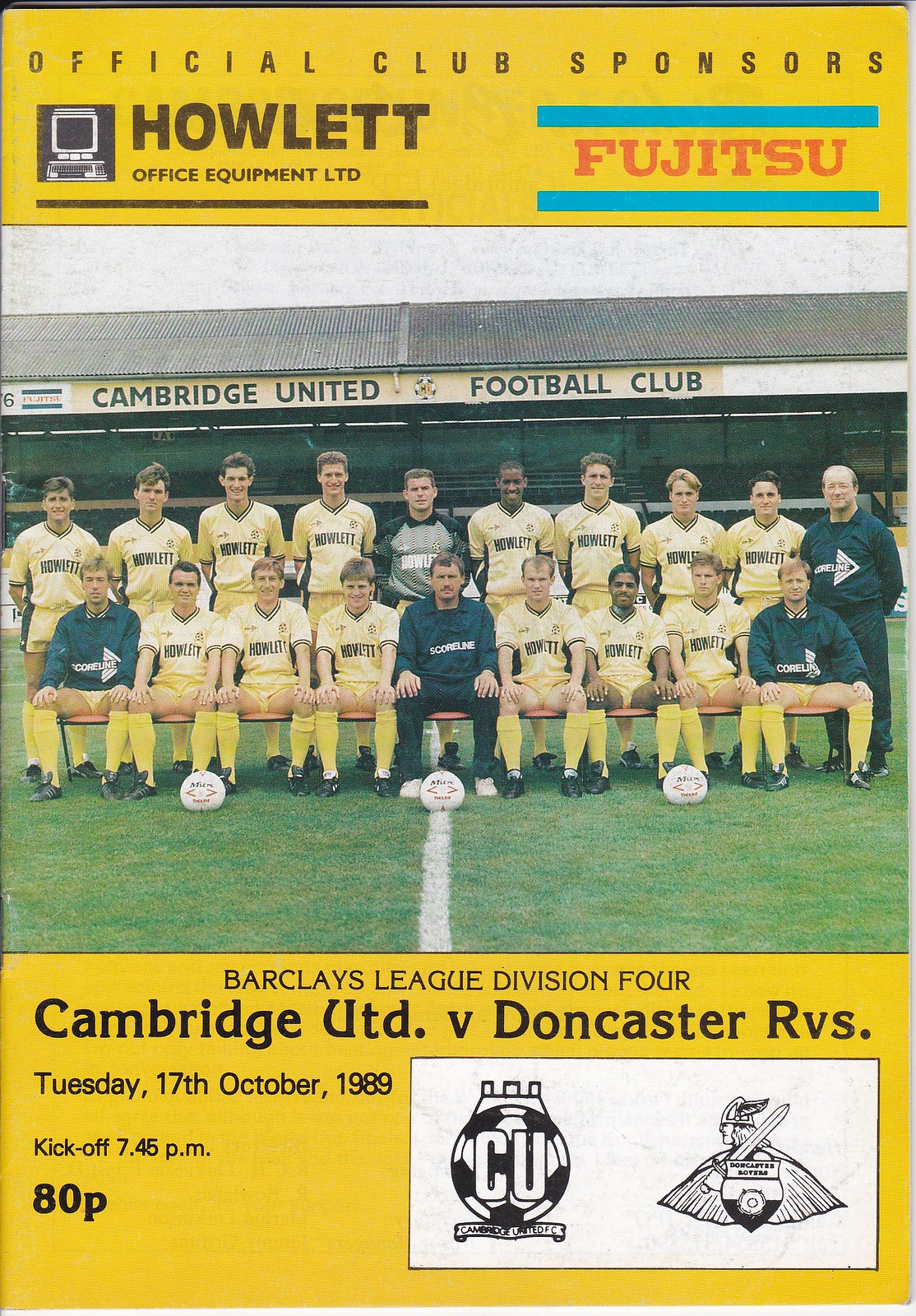This vertical goldenrod flyer is the cover for a soccer game program featuring Cambridge United Football Club. Across the top, it reads "Official Club Sponsors" in narrow black lettering. On the left side of the top golden bar, a logo for Howlett, Office Equipment LTD is displayed, featuring a black square with a white computer outline and the word "Howlett" in bold, sans serif font. To the right, "Fujitsu" appears in wide serif lettering, with bright blue horizontal bars framing the word. Below this is a large photograph of the Cambridge United soccer team, seated and standing in two rows on a green grass field. The front row is seated and wears white uniforms with gold-trimmed sleeves, yellow knee socks, and black athletic shoes, with three soccer balls in front of them. A coach in a black sweatshirt and pants is centered in the seated row. The background shows a stadium with a banner reading "Cambridge United Football Club." Below the photograph, the bottom golden bar displays "Barclays League Division IV" in serif lettering, followed by "Cambridge UTD v. Doncaster RVS," in bold serif font. To the left, in smaller font, it reads "Tuesday, 17th October 1989," and "kickoff 7.45 p.m. ADP." On the right side, two team logos are displayed: the Cambridge United logo, a black and white graphic of a soccer ball with "CU" inside, and the Doncaster logo, which features a winged warrior with a shield.